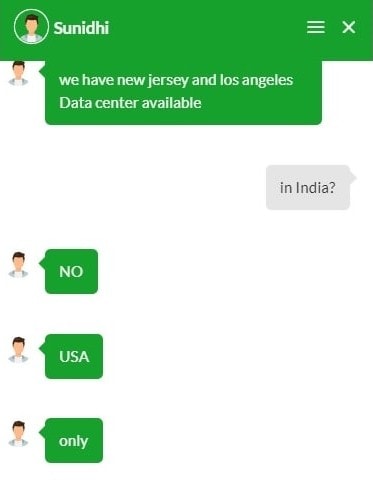This is a detailed screenshot of a mobile chat interface, likely part of a customer support exchange. The interface design, with its chat format and vertical dimensions, indicates it’s a mobile phone display. At the top of the screenshot, a green bar features an avatar of a faceless person in profile next to the name "Sunidhi". Adjacent to this is a three-bar menu icon and an 'X' button for closing the chat.

The chat conversation includes several exchanges. Sunidhi, the support representative, mentions that New Jersey and Los Angeles data centers are available. The user, responding in a gray speech bubble, asks, "in India?". Sunidhi replies emphatically with "NO" in capital letters, followed by "usa only" in lowercase letters. The responses from Sunidhi are aligned to the left side, while the user's messages are aligned to the right side. The image provides no additional context or details about the company or the specific nature of the support inquiry.